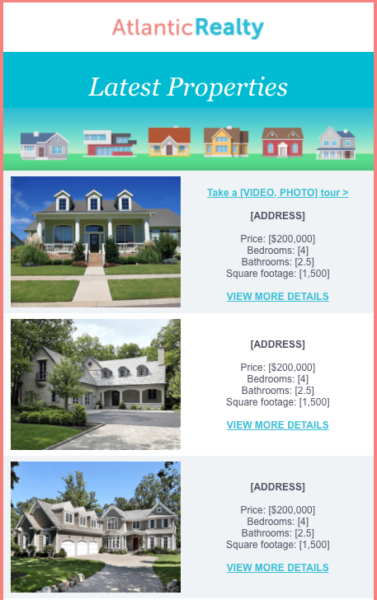The image depicts a real estate advertisement designed to look like a smartphone layout. The outer border of the ad is coral-colored, though the very bottom is not visible. 

At the top, there is a small white banner displaying "Atlantic Realty." The word "Atlantic" is in a light coral color, while "Realty" is in teal blue. Below this banner, there's another white banner with the italicized text "Latest Properties." This section features a panoramic view of a neighborhood consisting mainly of houses, all set against a backdrop of blue skies and greenery.

Further down, the ad showcases three property listings in a structured format:

1. **First Property**:
   - **Image**: A traditional house with three gables, a front porch, and a sidewalk running close to the lawn.
   - **Price**: $200,000
   - **Details**: 4 bedrooms, 2.5 bathrooms, 1,500 square feet.

2. **Second Property**:
   - **Image**: A similar or identical house in design.
   - **Price**: $200,000
   - **Details**: 4 bedrooms, 2.5 bathrooms, 1,500 square feet.

3. **Third Property**:
   - **Image**: Another house consistent in size and style with the previous listings.
   - **Price**: $200,000
   - **Details**: 4 bedrooms, 2.5 bathrooms, 1,500 square feet.

Each listing features a blue tab inviting viewers to "click for more details." Despite the uniformity in listed specifications and price, the houses visually appear as though they might differ in size.